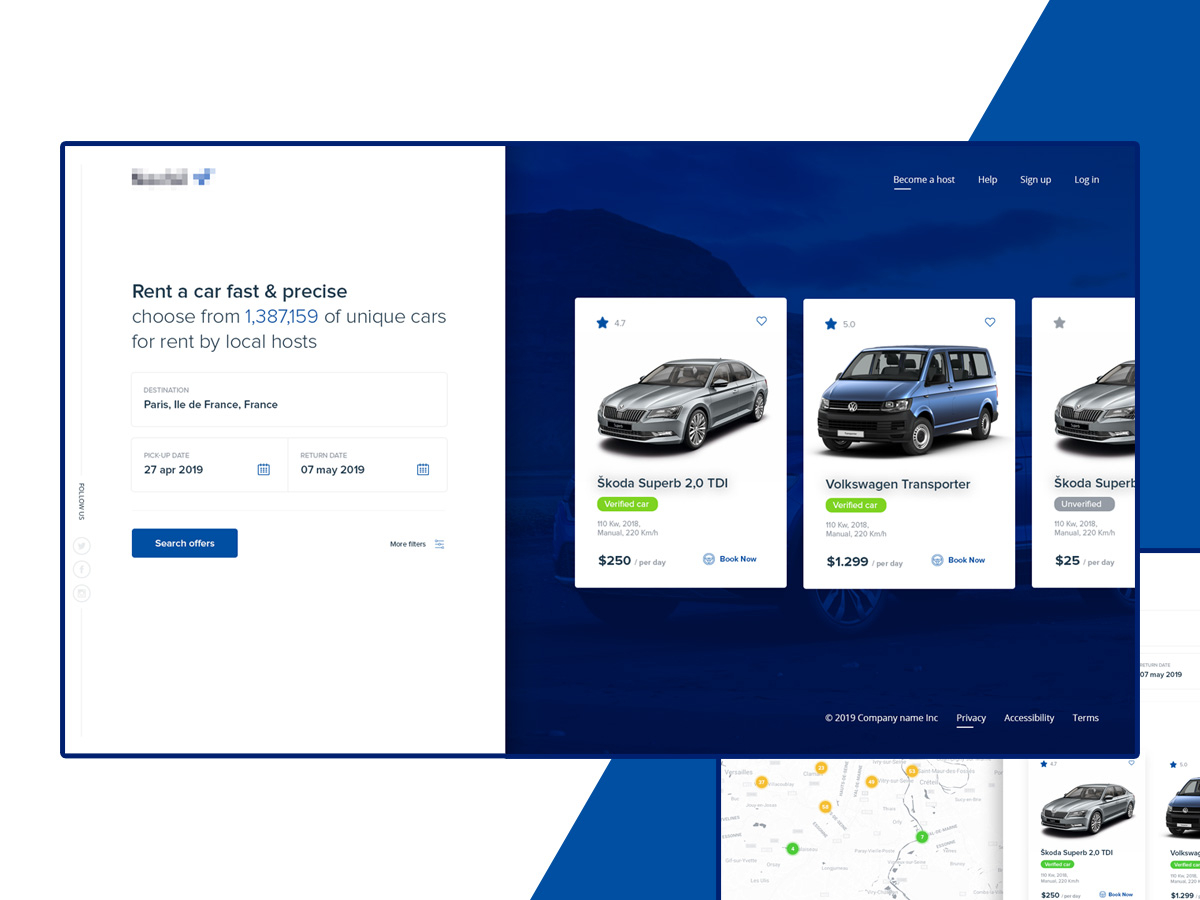The image depicts a web page with a predominantly white background, accented by a large blue section on the right side. Dominating the central part of the interface is a box outlined in blue, split into two sections: the left side is white, while the right side is blue. On the white section, there's a small, grayed-out spot with a tiny blue icon. The text within this box reads: "Rent a car fast and precise" in black font, followed by "Choose from 1,387,159 unique cars for rent by local hosts" with the numerical figures highlighted in blue and the remaining text in gray.

Below this, a white box contains the text "Paris, Ile-de-France, France," and another white box follows with the date "27 April 2019" accompanied by a small blue box. Another white box after this shows the date "07 May 2019," also paired with a small blue box. Adjacent to these date fields is a blue box with "Search offers" written in white. There is an additional white box, though its content is unclear.

On the left edge of the screen, several small icons and text snippets are visible. On the right side, set against the blue background, three car listings are displayed:

1. The first listing features an image of a car with one blue star and a heart, labeled as a Skoda Superb 2.0 TDI. There is a green tag indicating some special status, the price of $250 per day, and a "Read now" prompt.
   
2. The second listing shows a Volkswagen Transporter with one star and a blue heart. It includes a green box stating "Verified car," a price of $1,299 per day, and a "Book now" button.

3. The third car listing indicates a price of $25 per day. 

Underneath these primary listings, there is a small map, followed by details of two additional cars.